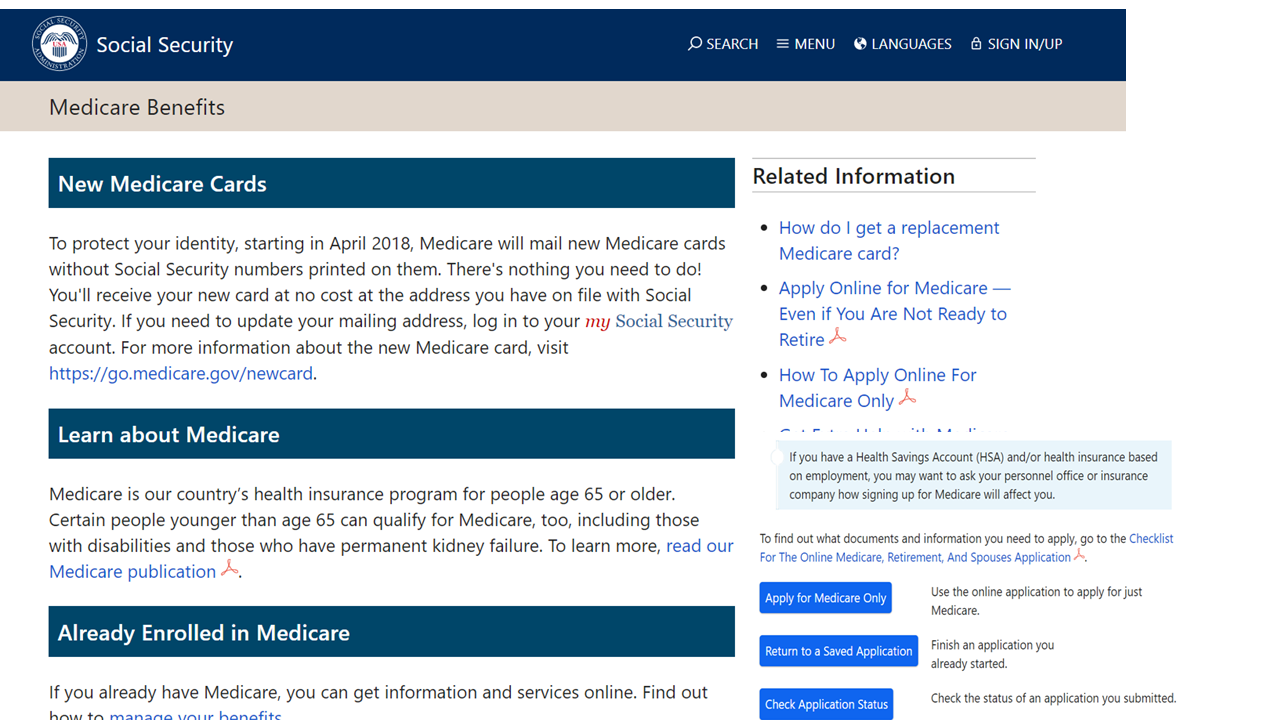The image depicts a webpage from the Social Security website, showcasing its organized layout and various sections. At the top of the page, a dark navy blue header features the official government logo of an eagle beside the text "Social Security" in white. This header also includes a search bar, menu option, language selection, and sign in/sign up option.

Beneath the header, a khaki-colored rectangular bar highlights Medicare benefits. Following this, several categories related to Medicare are prominently displayed. The first category focuses on new Medicare cards, detailed within a blue bar that includes a description and a URL link, "https://go.medicare.gov/newcard".

Further down, there is a section titled "Learn About Medicare", which describes Medicare as the nation's health insurance program. This section also includes a link to a Medicare publication, marked with the Adobe logo, suggesting it's a downloadable PDF.

Another section, "Already Enrolled in Medicare", also appears within a blue rectangular box. To the right of these main sections, there is a column featuring related information and various articles, each highlighted in blue, indicating clickable links.